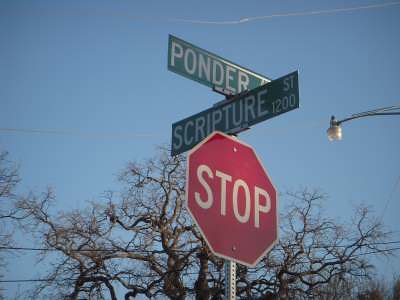This vibrant color photograph captures a vivid outdoor scene dominated by a prominent stop sign and two intersecting street signs mounted on a single, perforated silver pole. The street signs, a dark green with crisp white lettering, announce "Ponder" and "Scripture" at their respective intersections, with "Scripture Street 1200" clearly visible below "Ponder." The red, octagonal stop sign at the bottom of the pole features bold white letters and a white border. The background boasts a clear, cloudless, and bright blue sky, suggesting a beautiful sunny day. On the right side of the image, a street lamp curves into the frame, adding an element of urban infrastructure. Behind the street signs, leafless, gnarled branches of a tree stretch outward, indicative of a season when foliage is absent—likely winter, early spring, or late fall. Additionally, a few parallel power lines run across the scene, contributing to the urban landscape captured in this photo.